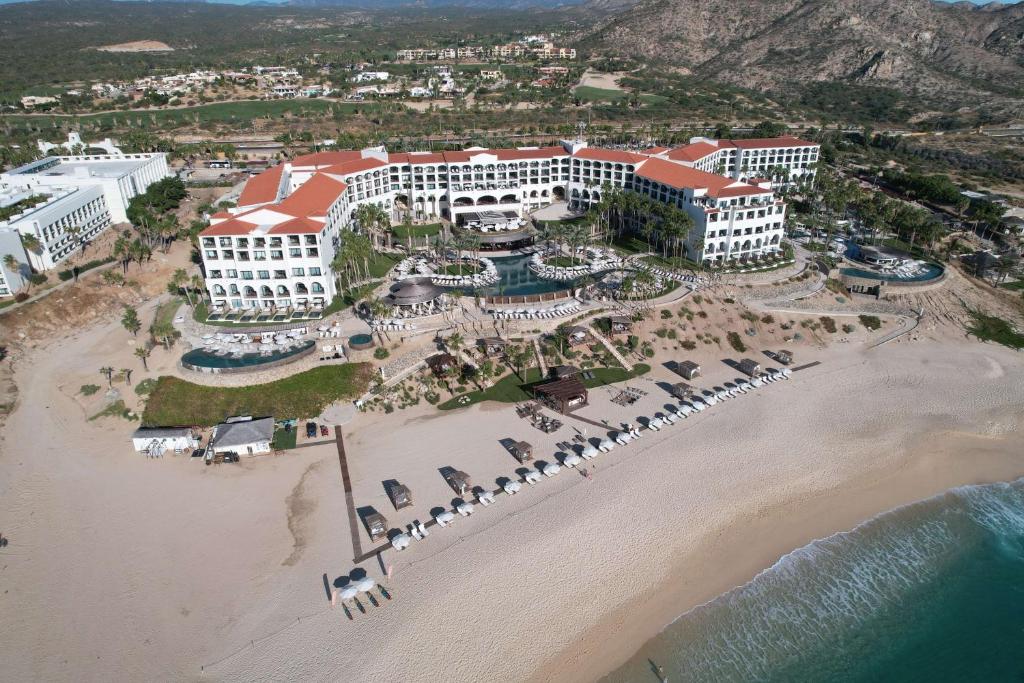This aerial photograph captures a stunning beachfront hotel resort situated on a sandy shore, with a large pool prominently featured in the front. The expansive, white U-shaped building, topped with a red roof, stands out as the focal point of the scene. Numerous beach tents and chairs are scattered along the tan-colored shore, offering a welcoming and relaxed vibe. The azure ocean waters create a striking contrast against the sandy beach, while the background reveals a lively cityscape interspersed with greenery, including lush grass and trees. The upper right corner showcases a rugged, gray and brown mountain range, adding a natural frame to this picturesque locale. The image is bathed in sunlight, emphasizing the bright, clear conditions of this beautiful outdoor setting.